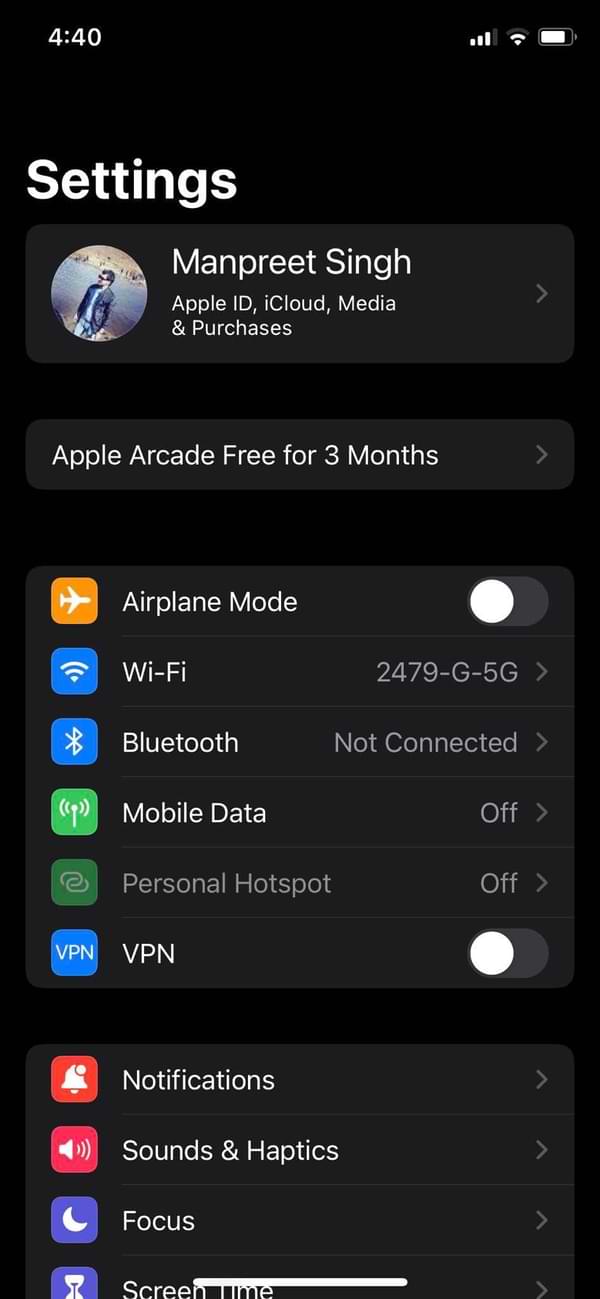A detailed screenshot of an iPhone's Settings screen captured at 4:40 PM. In the upper-left corner, the time is displayed, while the upper-right corner shows the Wi-Fi signal strength, cellular bars, and battery level. Below these system indicators, the main Settings menu is visible. At the top, the user's name is displayed along with options for Apple ID, iCloud, Media, and Purchases, each equipped with a clickable link for additional details.

Below the user's Apple ID section, there is a promotional banner offering three months of Apple Arcade for free, which also has a clickable link for more information. The Settings menu continues with several options: 

- Airplane Mode is currently turned off.
- Wi-Fi is connected to the network '24-79 G 5G.'
- Bluetooth is not connected.
- Mobile Data is turned off.
- Personal Hotspot is off.
- VPN is not enabled.

Further down, the menu includes options for Notifications, Sounds & Haptics, Focus, and Screen Time, each with a clickable arrow on the right to access more settings. The device is clearly in Dark Mode, as indicated by the dark background and white text. 

This is a comprehensive view of a typical iPhone Settings screen in Dark Mode.